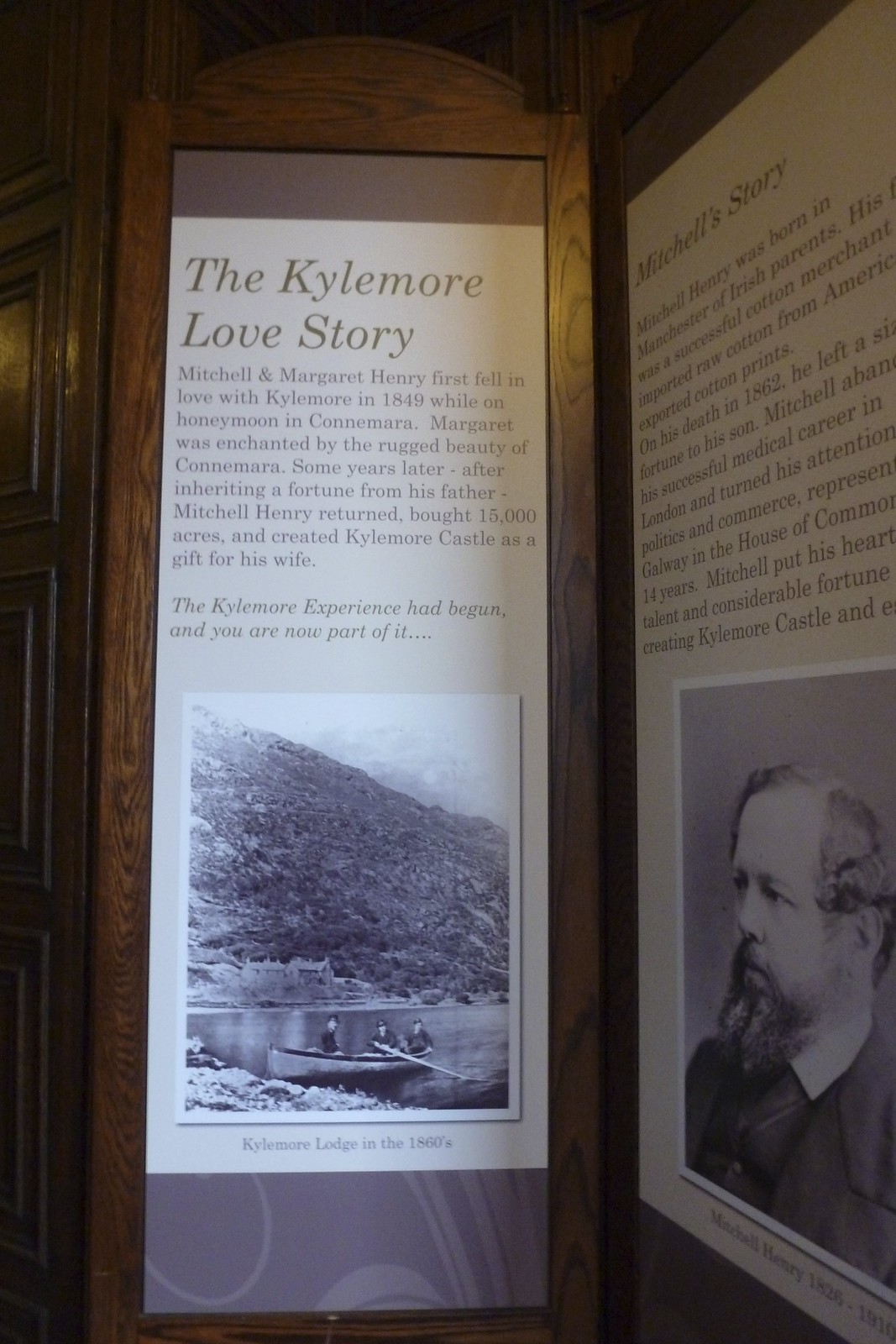The image showcases a wall inside an older building, possibly a museum or government structure, with rich wooden framing that displays informational posters. The left poster is titled "The Kylemore Love Story" in light gold lettering against a white background. It narrates how Mitchell and Margaret Henry first fell in love with Kylemore in 1849 during their honeymoon in Connemara. Margaret was captivated by the rugged beauty of the area, and years later, after inheriting a fortune, Mitchell bought 15,000 acres and built Kylemore Castle as a gift for her. Below this narrative, a black-and-white photograph depicts three individuals paddling a canoe on a lake, with a bushy hillside and distant mountains in the background, labeled "Kylemore Lodge in the 1860s."

On the adjacent wall to the right, another poster, titled "Mitchell Story," is harder to read due to the angle of the photo but features a portrait of Mitchell Henry, an older man with mottled gray hair, a dark beard, and a mustache, dressed in a dark suit with a stiff white collar. This photo likely captures more details about the builder of Kylemore Castle, highlighting his contributions and legacy. A wooden door is visible beside the poster, reinforcing the historical ambiance of the setting. The entire layout suggests that the photograph was taken by a visitor using a cell phone, capturing a moment of discovery inside a room dedicated to the history of Kylemore Castle and its creators.